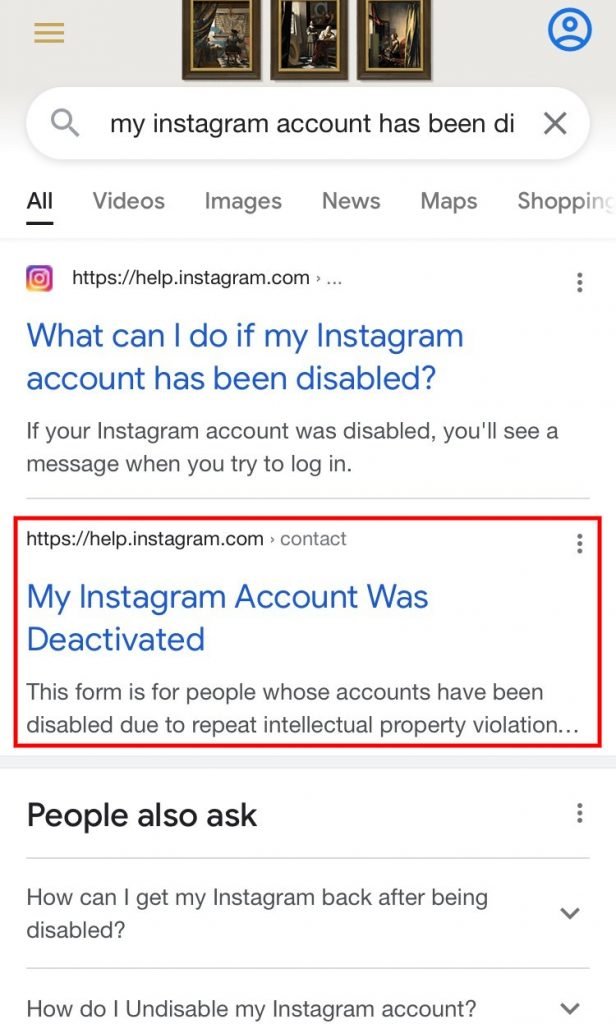This image is a screenshot, seemingly taken in portrait mode from a mobile device. The interface is likely a web browser or a documentation app, given the layout and elements visible.

The upper section of the image features a dark cream background, with three horizontal gold lines on the upper left corner, presumably representing a menu icon. Centered at the top are three framed artistic oil paintings, though their significance isn't clear from the text alone. On the upper right corner, there is a blue circular icon resembling a user account icon.

Directly underneath this top bar, there is a search bar containing the text, "my Instagram account has been DI." Below the search bar are category headers, including "All," "Videos," "Images," "News," "Maps," and "Shopping," with "All" being underlined, indicating it is the selected category.

The first search result displayed is from help.instagram.com, identified by the Instagram icon. The link reads, "What can I do if my Instagram account has been disabled?" in blue text, followed by a brief explanation: "If your Instagram account was disabled you'll see a message when you try to log in."

Below this, the next row features a prominently marked section, highlighted in red by the person who took the screenshot. This result originates from help.instagram.com and includes the blue text link, "My Instagram account was deactivated." It further details, "This form is for people whose accounts have been disabled due to repeat intellectual property violation."

The bottom of the screenshot shows three questions under the "People also ask" section: 
1. "How can I get my Instagram back?"
2. "How do I un-disable my Instagram account?"

The overall context of the image suggests it is a part of a guide or search results on how to address issues related to a disabled Instagram account.